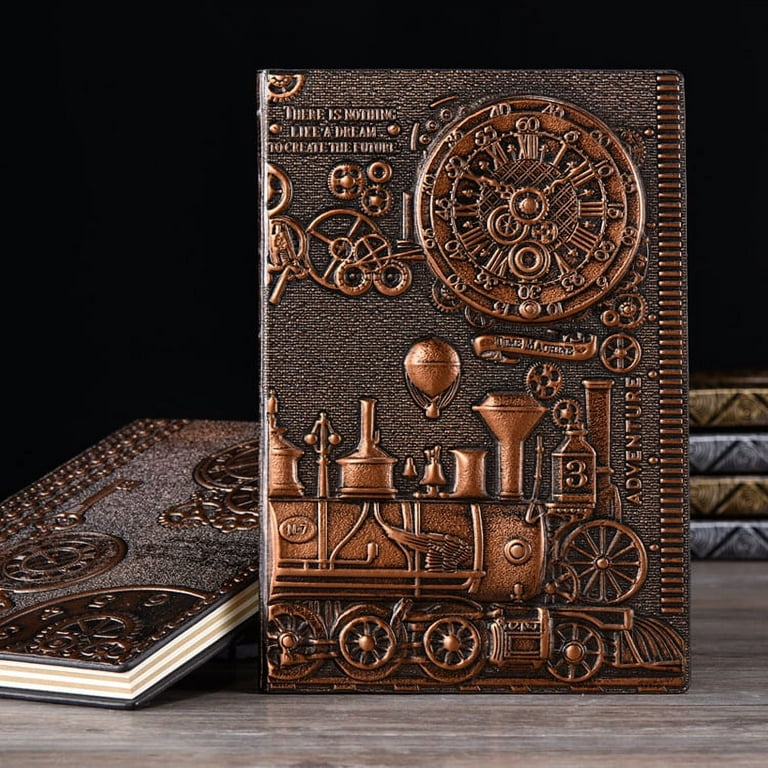The image depicts an assortment of antique-looking journals, each adorned with elaborate, metallic steampunk designs. The central journal, prominently positioned facing the viewer, features a cover with intricate brass, copper, and brown tones, evoking a vintage aesthetic. The cover showcases an array of mechanical elements, including a prominent clock with gears and screws cascading to the ground, a classic steam engine with ornamental wings, and a hot air balloon. The upper left corner bears the inspirational text, "There is nothing like a dream to create the future," embossed in raised lettering. Below the clock, there's a ribbon inscribed with "Time Machine," and the word "Adventure" is etched along the side. Surrounding this focal journal are several other journals, some stacked in the background and another lying flat, all sharing a similar metallic, clockwork motif. The scene is set against a wooden table and a dark backdrop, enhancing the aged, steampunk ambiance of the image.